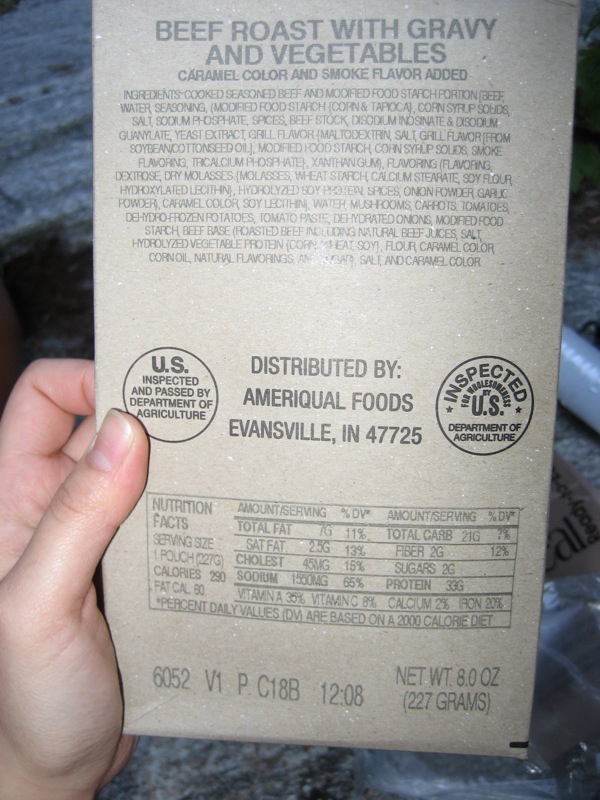In this close-up photograph, a white person's left hand holds a gray-brown roast beef with gravy and vegetables packet against a backdrop of a purple blanket. The packet prominently features the text "Beef Roast with Gravy and Vegetables" at the top, followed by "Caramel Color and Smoke Flavor Added." The densely packed ingredient list covers one-third of the image. Centered on the packet is the distribution information: "Distributed by Ameriqual Foods, Evansville, IN 47725." Flanking the distributor details are circular stamps reading "U.S. Inspected and Passed by Department of Agriculture." Below these stamps, nutritional facts are printed, indicating a net weight of 8 ounces. The text appears gray against the brown cardboard material, contributing to its hard-to-read nature.